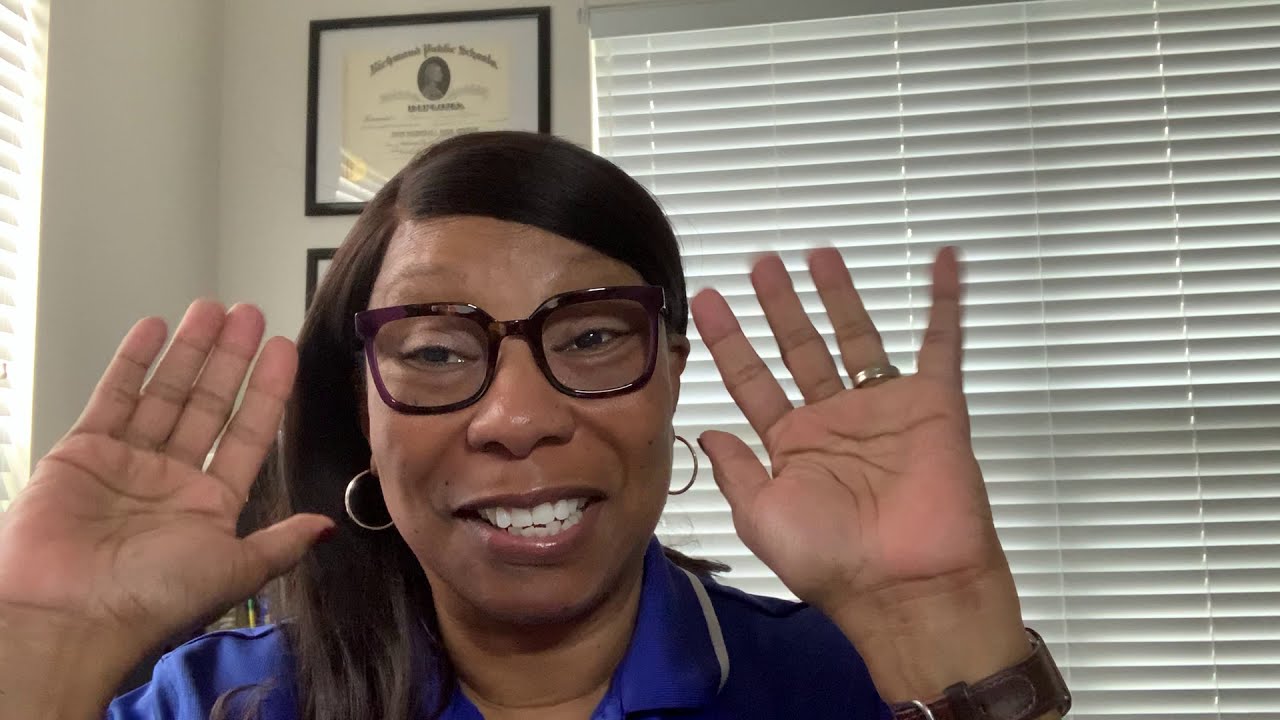The image features Sophie, a woman with light brown skin and long, dark brown straightened hair. She is smiling warmly at the camera, which causes her eyes to squint. She wears dark purple glasses with large rims and two silver hoop earrings. Sophie is dressed in a blue outfit that appears to be a medical or nurse's uniform. She has a ring on her right hand and a watch on her right wrist. Her hands are raised beside her face, palms open. Her face has a couple of distinguishing moles, one on her cheek and another just above her mouth. The background suggests she is in an office or home office environment, as there are white walls and white blinds covering the windows on both the right and left sides of the image. Behind her, on the right side, black photo frames with certificates are hanging on the wall, though they are too blurry to read. A subtle light filters through the blinds, illuminating the room, which also contains a desk with some visible office supplies like pencils.